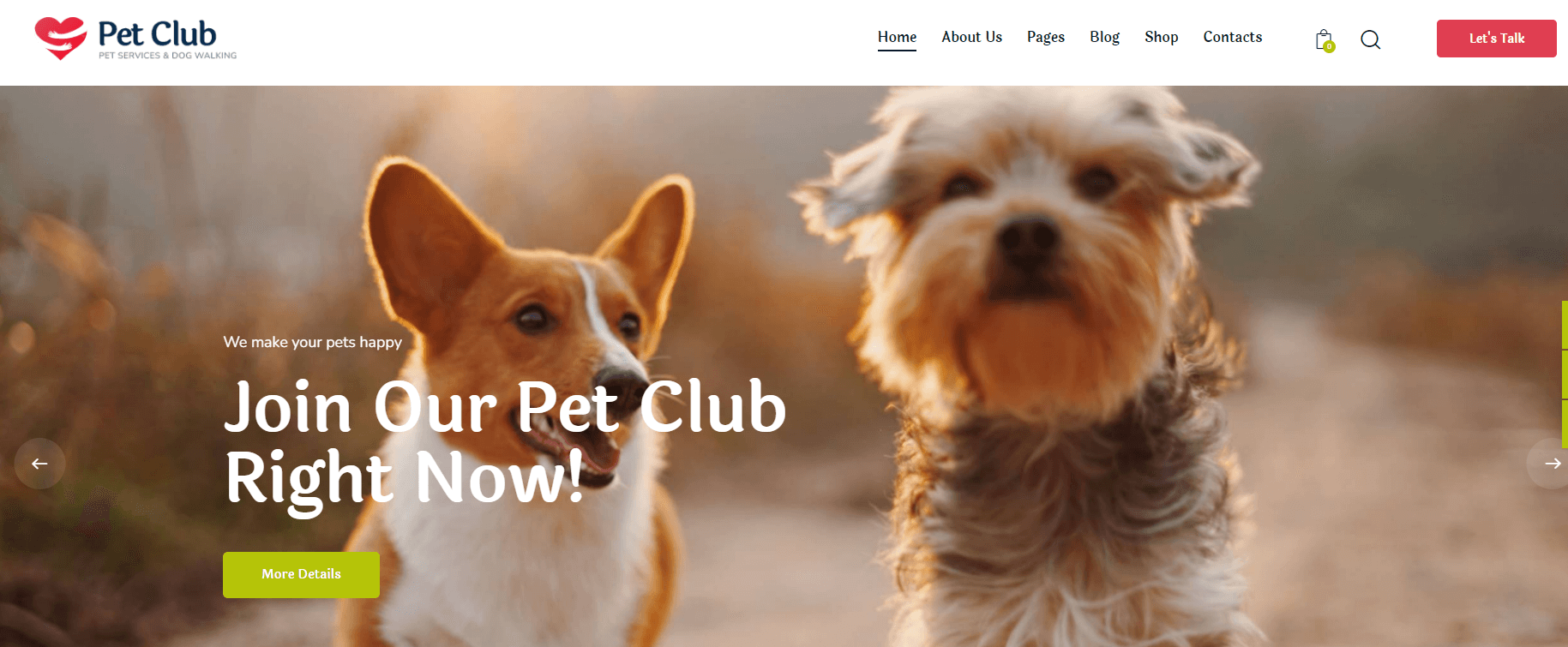**Website Homepage Overview**

At the top of the website, there is a charming logo featuring a heart with two small white arms gently wrapping around it, reflecting love and care. Adjacent to the logo, the website title "Pet Club" is prominently displayed. Directly across the top navigation menu, visitors will find options such as "Home" (which is underlined), "About Us," "Pages," "Blog," "Shop," and "Contacts." To the right of the menu, there is a search icon in the shape of a magnifying glass and a striking red button labeled "Let's Talk."

**Hero Section**

Beneath the navigation, a warm and inviting call-to-action image takes center stage. The image contains the words, "We Make Your Pets Happy, Join our Pet Club Right Now," accompanied by a gold button that says "More Details." The background of the image is intentionally blurred, drawing focus to the foreground where two adorable dogs are standing side by side.

**Dog Descriptions**

In the foreground, the focus is on a cute yorkie, which appears to be very close to the camera, giving the impression that its nose might boop the screen. The yorkie showcases its typical brown, white, and black fur, although its ears are intriguingly down, suggesting it might not be a full yorkie. Its expressive brown eyes and endearing nose contribute to its cuteness.

Next to the yorkie stands another dog that looks somewhat like a corgi. This dog has a distinctive brown face with a wide white stripe running from its nose up to its forehead, complemented by a large white chest. Together, these dogs create an irresistible image, perfect for evoking the playful and tender sentiments associated with pet companionship.